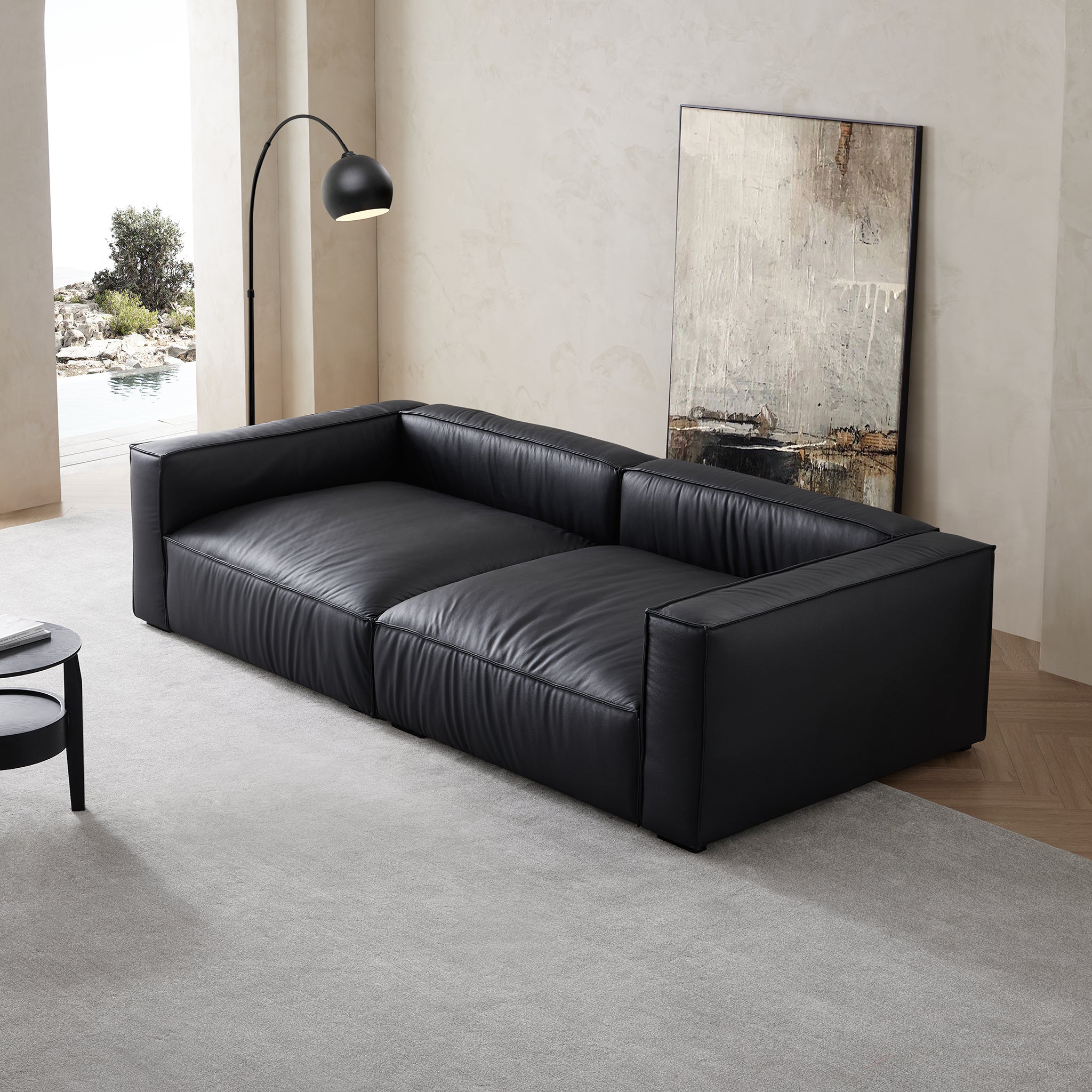The image depicts a modern, minimalist living room with a sleek, black leather-like lounge sofa featuring two oversized square cushions, low arms, and a low back. The sofa is centered on a light gray area rug that partially covers a chevron-patterned light wood floor. Behind the sofa, leaning against a beige Venetian plaster wall, is a large abstract painting in tones of beige, gray, black, and brown. To the left of the sofa stands a black metal reading lamp with a dome-shaped shade, arching gracefully over the sofa. A doorway on the left side of the room opens to an outdoor space with a pool and surrounding greenery.